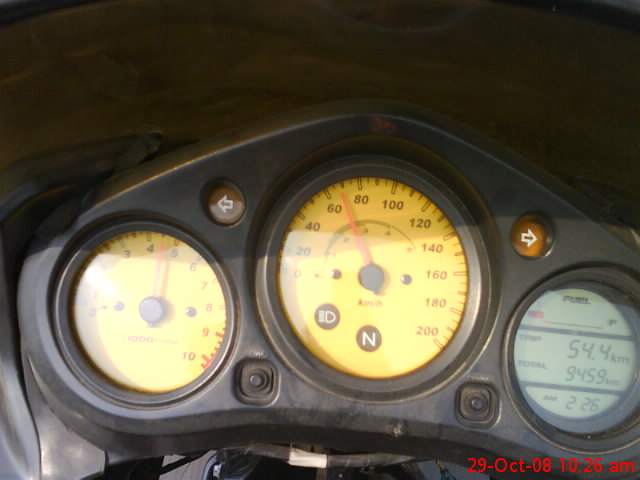A photograph taken on October 29th, 2008, at 10:26 a.m. showcases the control panel of a motorbike. The control panel design features a slightly triangular point at the top transitioning to a gently concave bottom edge. Central to the panel are three circular bezels. The middle bezel houses a yellow speedometer that measures up to 200 kilometers per hour. The panel includes an emblem indicating the status of the headlights and another at the bottom for neutral gear indication. On the left side of the panel is a yellow RPM gauge numbered 1 through 10, while on the right, a white-background fuel gauge allows the rider to monitor the fuel level. The contrast between the yellow and white gauges ensures easy readability for the rider.